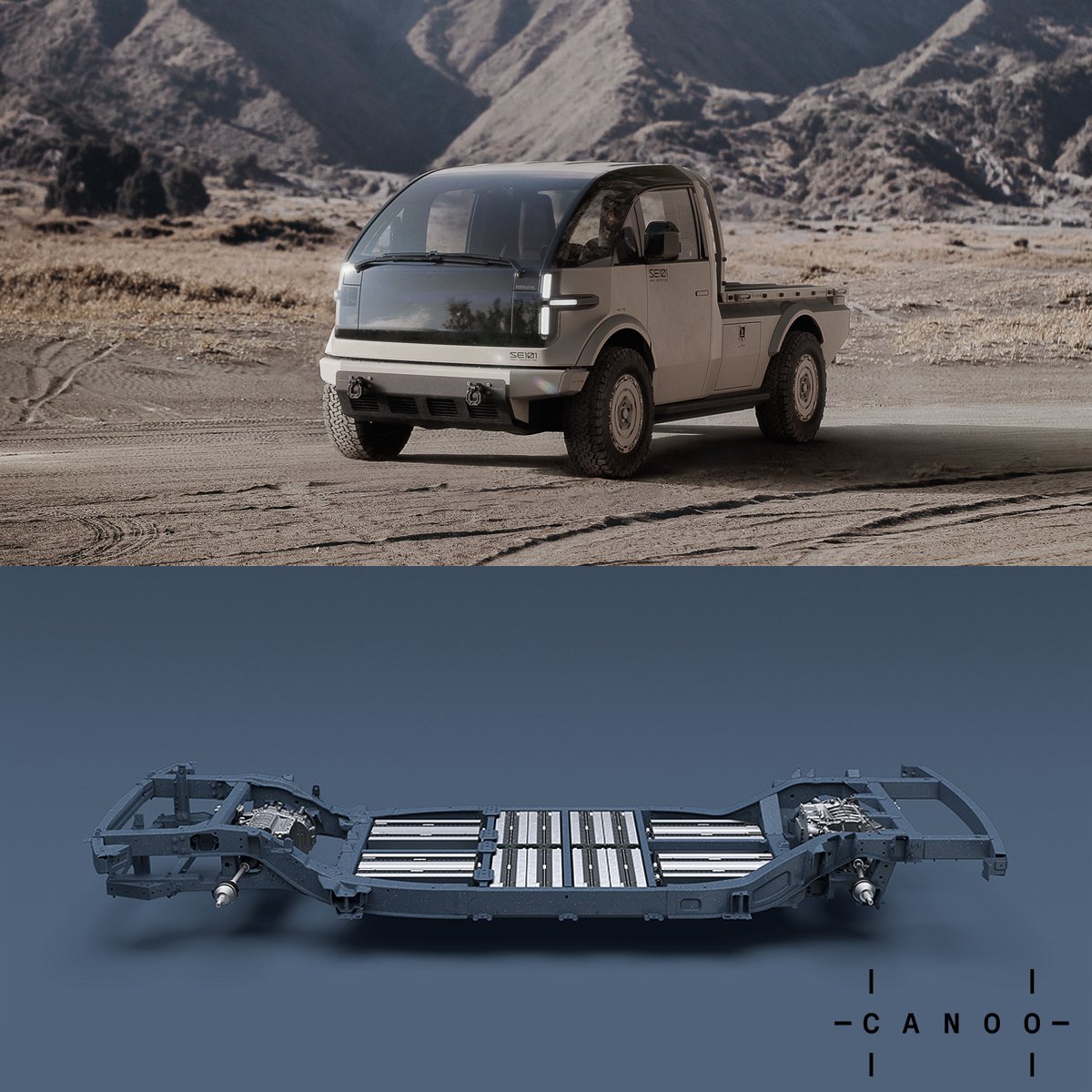This detailed image captures a futuristic electric pickup truck by Canoo, presented in two main sections. The upper part of the image showcases the sleek, off-white truck navigating through a rugged, desert-like environment with rocky mountains and sparse, dried vegetation in the backdrop. The truck features a unique, aerodynamic design with a smooth, glass-domed front, large curved windows, and a small rear bed, riding on four black wheels. The image's dramatic, extraterrestrial-like landscape adds to the vehicle's avant-garde appeal.

The lower part of the image reveals the truck's chassis against a blue background, highlighting its electric powertrain. The chassis is predominantly dark blue with silver battery packs, black lines, and two robust axles housing silver motors. This close-up gives a clear view of the vehicle’s underpinnings, emphasizing its electric nature.

In the bottom right corner, the company's logo, "Canoo," is displayed prominently, with artistic dashes surrounding the "C" and the "O." This comprehensive image effectively portrays both the futuristic exterior and sophisticated internal components of Canoo's innovative electric truck.